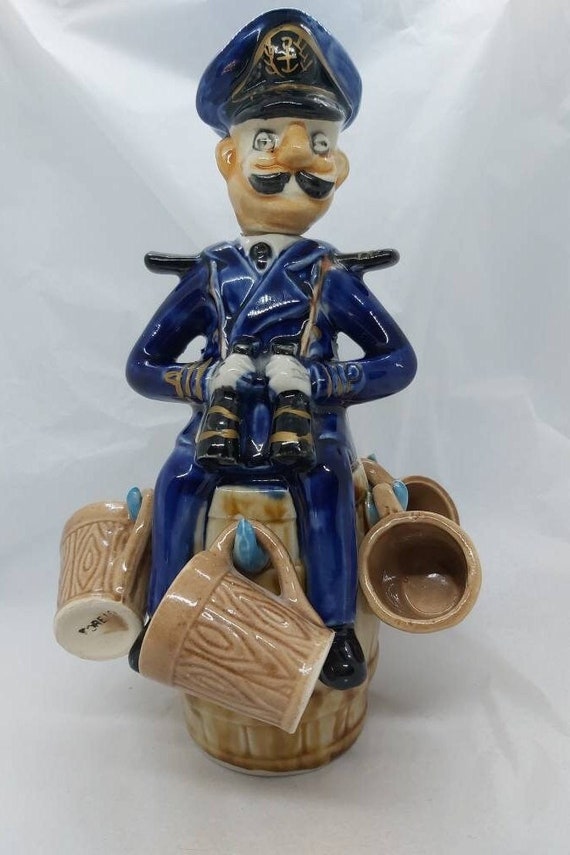This detailed and vibrant photograph captures a vintage porcelain figurine of a sea captain, likely from the 1940s or 1950s, featuring intricate craftsmanship. The captain, depicted as a white man, is elegantly attired in a blue sailor’s suit with white gloves, and a blue-and-black seafaring hat adorned with a gold-trimmed anchor emblem. His distinguished appearance is enhanced by a large, fruffy mustache and a pleasant smile on his tan face. Seated on a rustic brown wooden barrel, the captain clutches binoculars in his white-gloved hands, embodying a navigational pose. The barrel itself is a central element, equipped with blue hooks that support several wooden mugs or shot glasses. The entire scene is set against a backdrop that appears to be a crumpled piece of light gray or white cloth, adding a textured, antique ambiance to the overall composition.